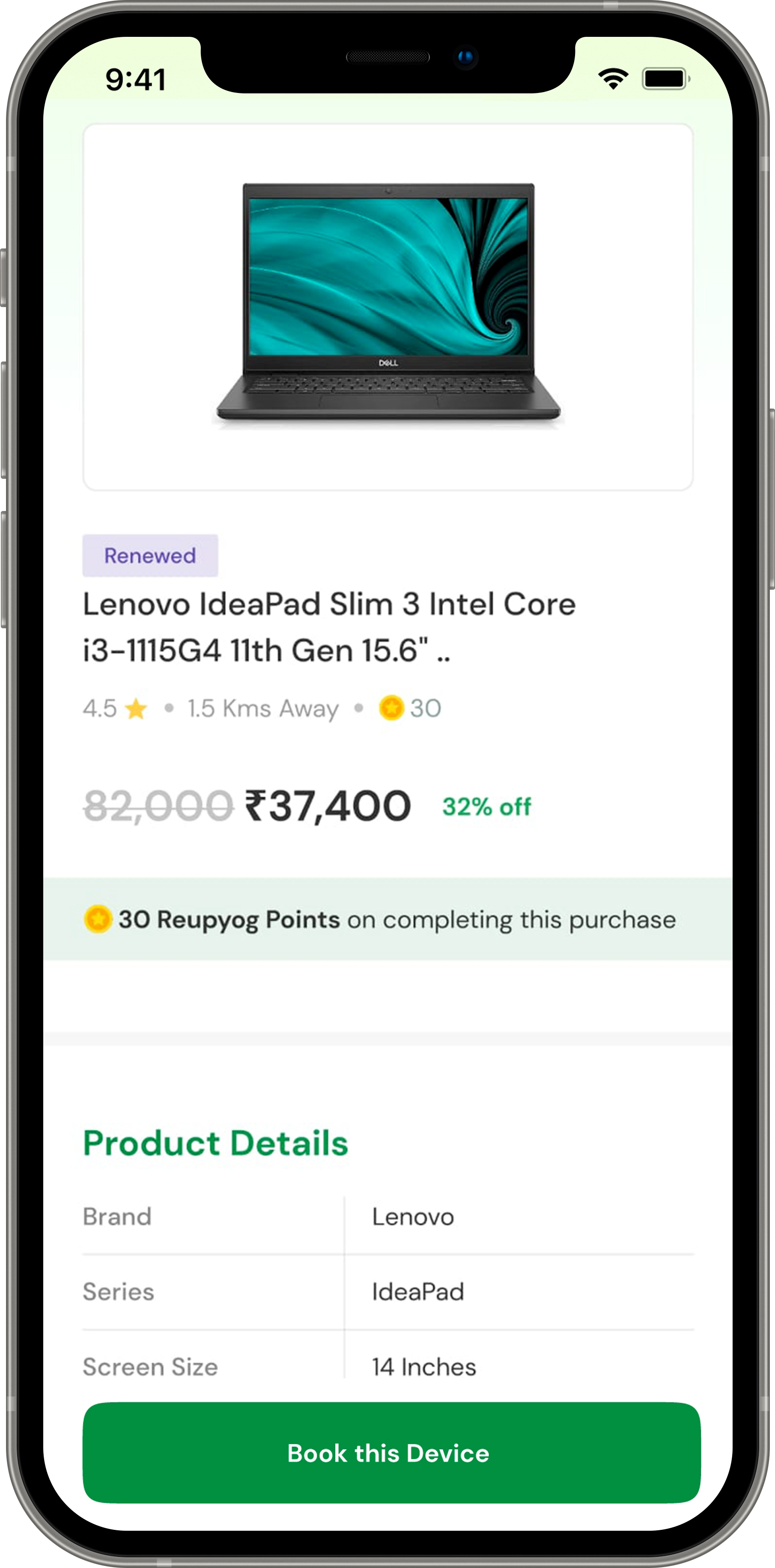Here is a cleaned up and detailed caption for the described image:

----

The image is a stylized graphic of a mobile phone with a sleek design, featuring a black border and a thin silver exterior. The phone has three buttons on the left side and one button on the right side. The screen displays a time of 9:41 and has a light greenish-gray background. At the top of the screen, there's an image of an open black laptop with a dark bluish-green swirl as its screensaver. Below this, there is a gray box with the text "Renewed" in purple. Underneath, details about the laptop are provided in black text: "Lenovo IdeaPad Slim 3, Intel Core i3-1115G4, 11th Gen, 15.6". The laptop has a rating of 4.5 stars and is 1.5 kilometers away from the user's location. The price has been reduced from $82,000 to $37,400, offering a 32% discount. Additionally, the purchase includes 30 Reupyog points, spelled R-E-U-P-Y-O-G. At the bottom of the screen, there are some product details and a button labeled "Black Book List Device".

----

This caption is detailed and provides a clear description of the image and its contents.